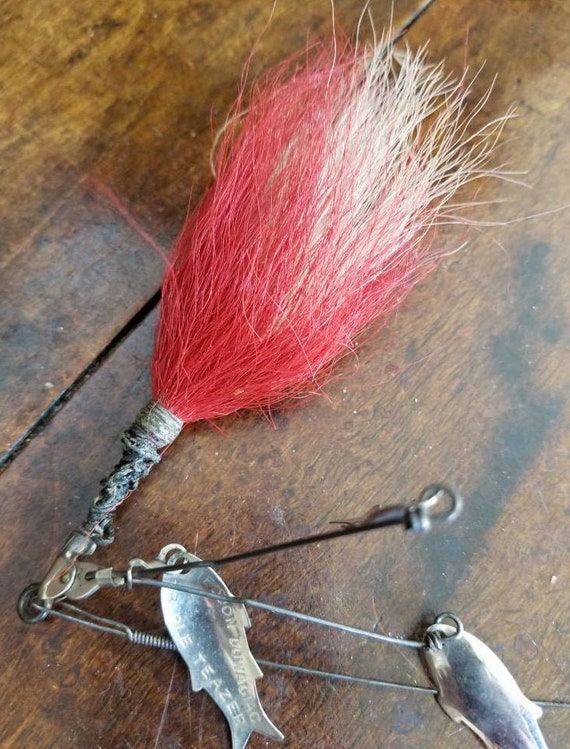This is a close-up photograph of an antique fishing lure, lying on a dark wooden table. The lure features a distinctive, brush-like tail made of red and pink hair with occasional white strands. This colorful, fur-like material is attached to a black metal rod with a rusted gray tip. Extending from the rod are two small silver fish, designed to spin or swim through the water to attract other fish. One of the fish is engraved with the words "triple teaser" and is turned over, revealing the inscription, while the other lies right side up, obscuring its text. The lure appears well-worn and rustic, indicative of its age and use in fishing.